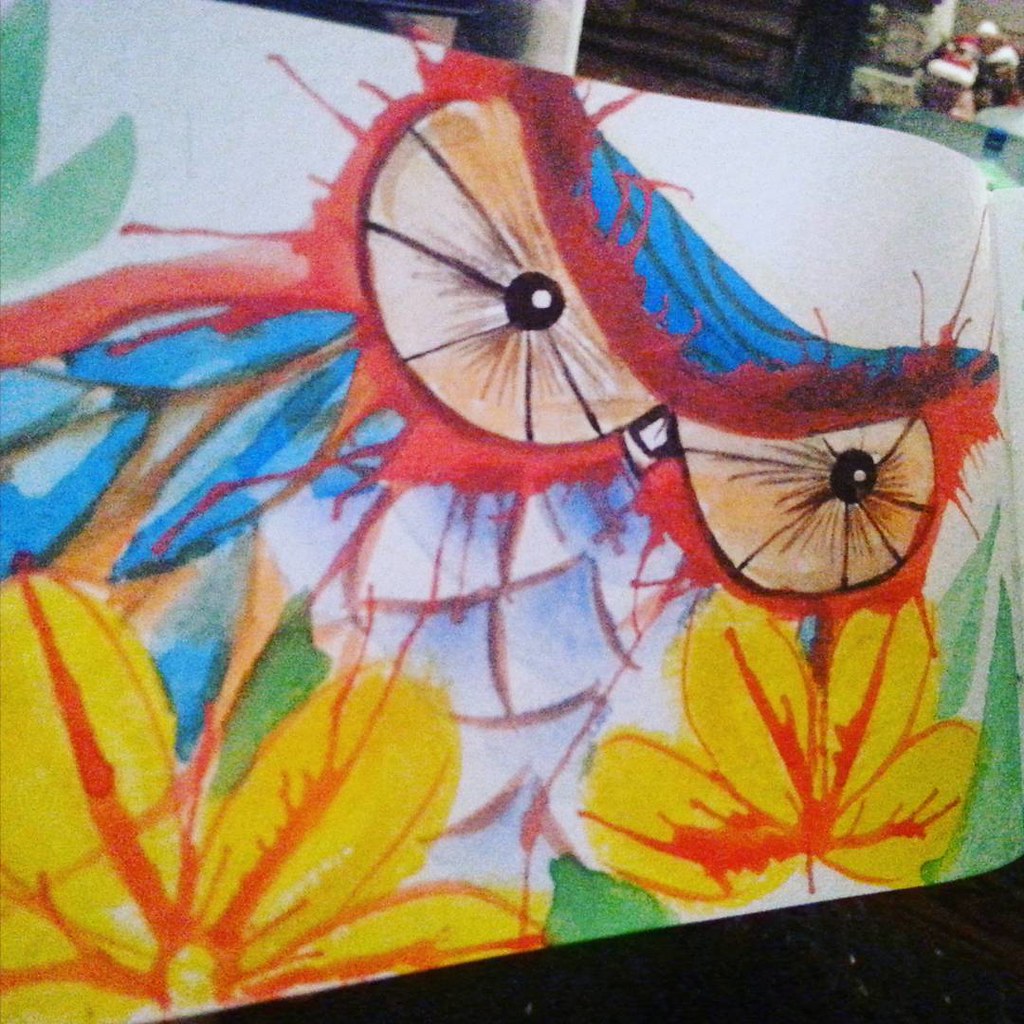The image is a photograph of a watercolor painting on a white paper or canvas, set in a room with a visible shelf in the background. The painting depicts an owl with striking, expressive features. The owl has a blue head and blue feathers, with lighter blue on its chest. Its eyes are particularly vivid, rimmed in red paint that extends outwards in wispy, feather-like patterns. The eyes are tan with black pupils, accented with black lines and white highlights that give them a shimmering effect. The beak is white, outlined in black, adding to the owl's intense gaze.

In terms of additional details, a variety of design elements frame the owl. There are blue leaves on the left and right, along with green leaves in the top left and bottom right corners. The background also features yellow and orange leaf designs, as well as yellow flowers near the bottom. Red hues are present throughout the painting, particularly around the owl's eyes and in its wings. The mix of colors and intricate designs, including what appear to be scales, contribute to a rich and dynamic composition. Overall, the painting might come across as an amateur artwork, but its detailed and vivid depictions evoke the image of an owl amidst a natural setting.